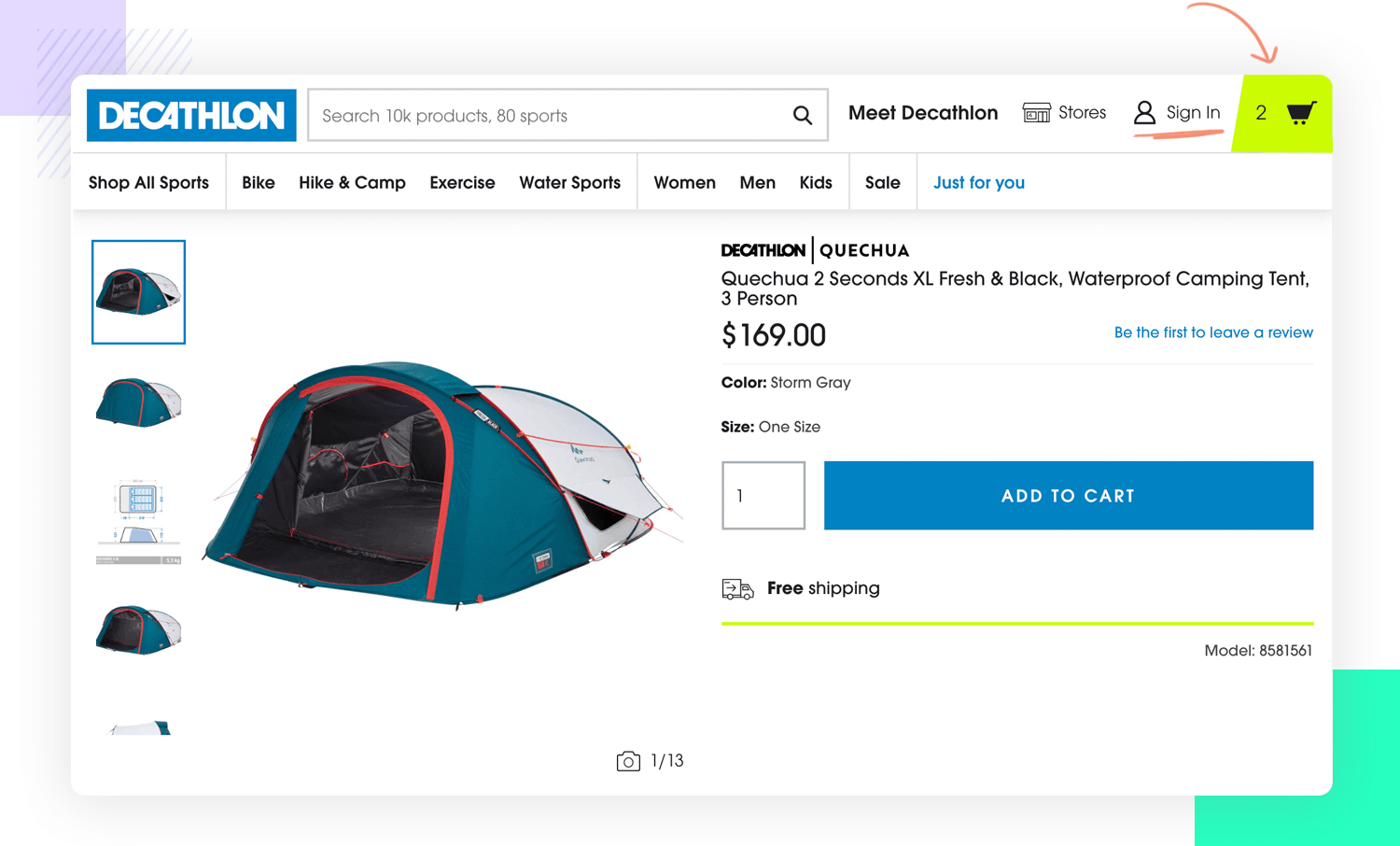This is an elaborate screenshot of a Decathlon store’s online shopping page, showcased in a horizontally rectangular format positioned in the upper left corner of the screen. The background features a lavender-colored square with a smaller, gray diagonally striped square overlaying the right half of it. Additionally, a green square is partially obscuring the lower right portion of these squares. 

The website interface prominently displays a search bar with the text "Decathlon Search 10k products 80 sports." Adjacent to this, towards the right, is the “Meet Decathlon” section, accompanied by a building icon and a prompt to find stores. Further to the right is a sign-in icon. On the far right end of the header, there is a shopping cart icon with the number 2 displayed to its left, housed in a green, angled square. A red, curved arrow points downward towards the shopping cart, highlighting it.

The featured product on this page is a blue, red, and white tent pictured on the left side of the screen. The detailed description on the right side reads "Quechua 2 Seconds XL Fresh and Black Waterproof Camping Tent 3 Person" priced at $169. The color is noted as ‘storm gray,’ although the displayed color does not appear to be gray. The listing also mentions that the item comes with free shipping.